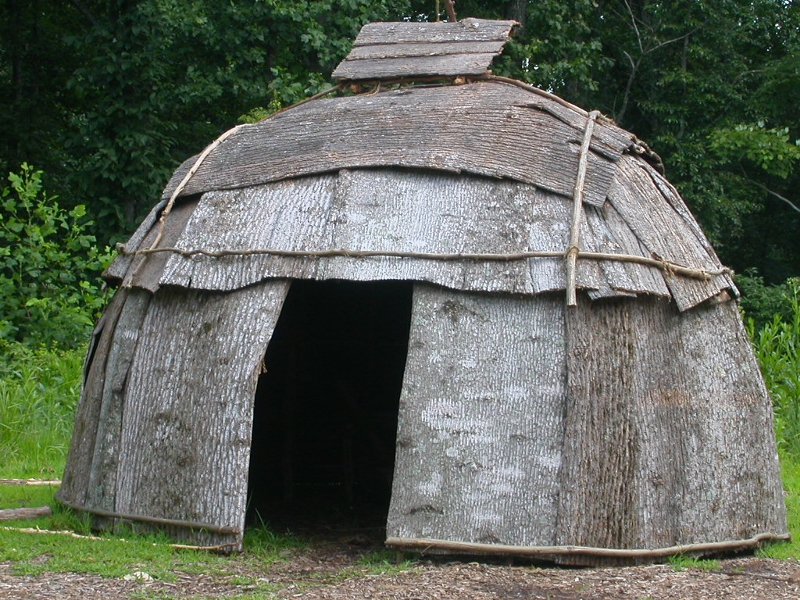This photograph showcases a large, distinctive wooden hut situated in the heart of a jungle. The structure exudes a helmet-like, oval shape, predominantly grey in color, constructed meticulously using sticks and bark from trees. Its central square door leads into a dim interior, with a ladder faintly visible in the backdrop. The hut stands approximately eight to nine feet tall, with an additional foot or two allocated to its unique slanted A-frame roof, which is capped by what appears to be a chimney. The ground surrounding the hut is primarily dirt, contrasting with the lush greenery of grass, shrubs, and an array of trees that populate the background. The dome-like structure of the hut, reinforced by wooden framing, positions it prominently at the center of the image, offering a vivid display of rustic architecture harmonized with its verdant jungle setting.